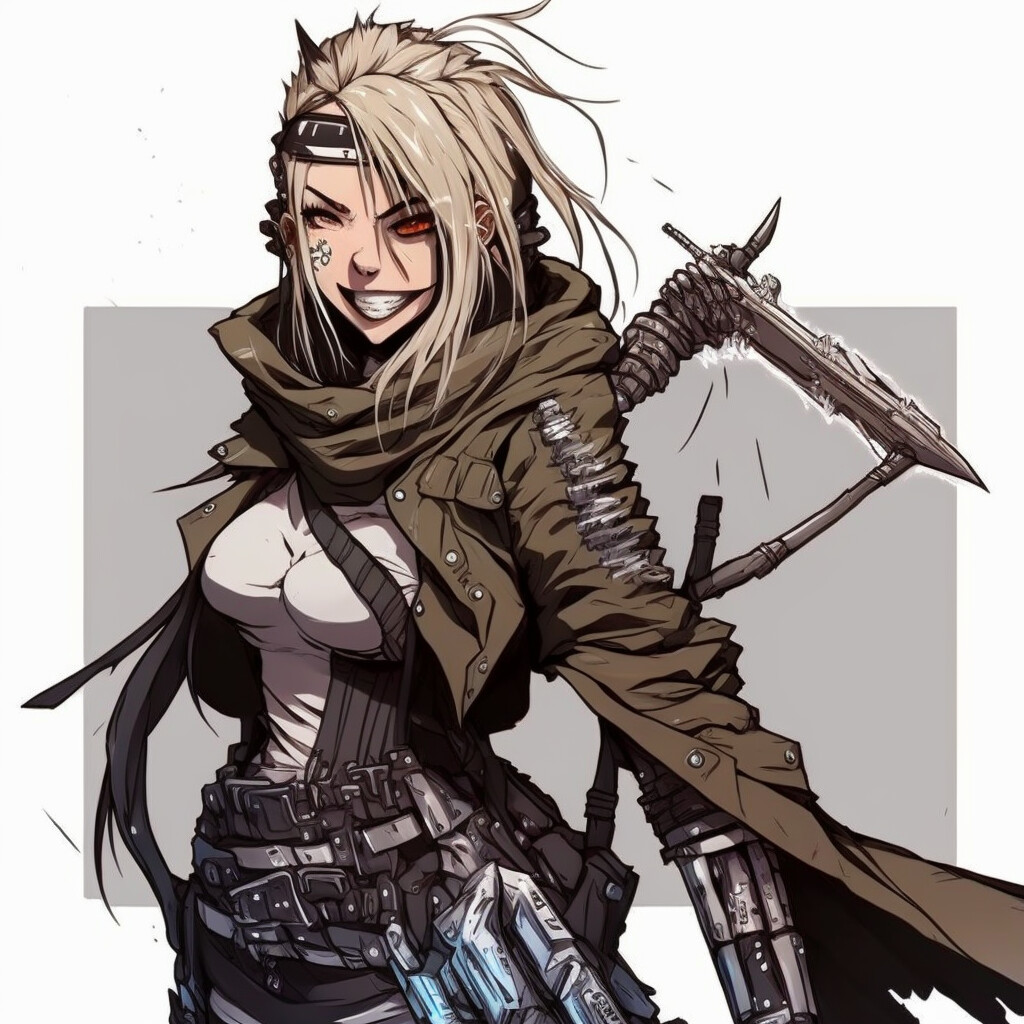This image features a striking female warrior, clearly inspired by video games or anime. She has long, spiky blonde hair and wears a black headband across her forehead. Her eyes are distinctively different: one is a glowing, eerie red, while the other is a normal brown or hazel. Her facial features include a triangular-shaped, devious smile and a noticeable tattoo or marking on her right cheek.

She is dressed in a brown, shawl-like jacket or trench coat that flows around her neck, complemented by an off-white, tight tank top that accentuates her pronounced bust. Her left arm appears mechanical and features white markings, contrasting with her otherwise human form.

Various weapons are strapped to her body: a menacing crossbow or blade is holstered on her back, while her waist is adorned with multiple belts holding tools, ammunition clips, and additional weapons. Her attire, combined with her warrior-like appearance and the arsenal she's carrying, firmly plants her character in the realm of anime or action video games.